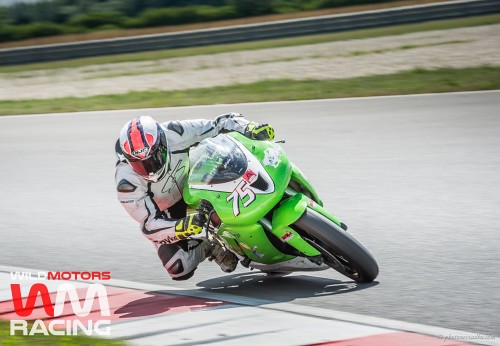This color photograph captures a motorcyclist racing on a lime green motorcycle, which is almost tilted entirely on its side, indicating high speed. The rider is adorned in a white protective suit with black designs, complemented by knee pads and yellow and black gloves. His helmet is white with an orange design and features a black visor. He is deeply crouched over the front of the bike, leaning aggressively to the left, highlighting the intensity of the corner he's navigating on a paved racetrack surface. In vibrant contrast, the track markings at the corner are painted red and white, with grassy areas and a tan wall in the distance. The scene, set in early evening with daylight still visible, shows the horizon line with some trees in the top left corner. Notably, the bottom left corner of the image features the logo for WM Wild Motors Racing, with the "W" in red and the "M" in white above the word "Racing" in white, subtly tying the thrilling action to its racing team.